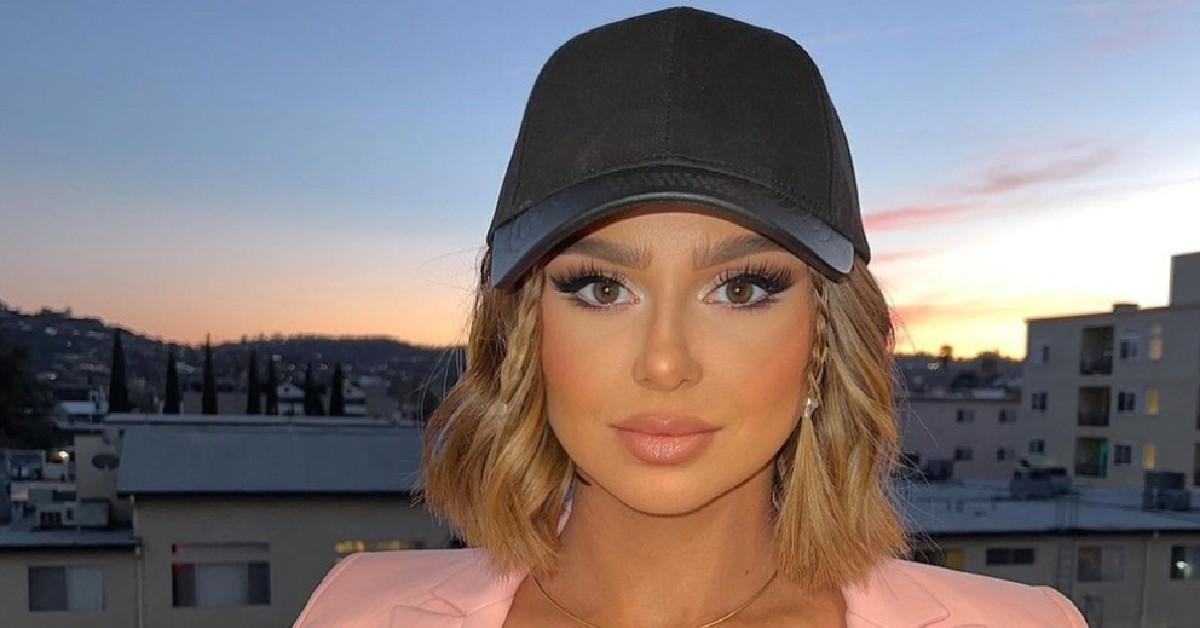In the close-up photograph of a Caucasian woman looking directly into the camera, she is adorned with a black leather baseball cap and her shoulder-length, wavy blondish-brown hair features two thin braids framing her face, each embellished with tiny jewels. Her makeup is meticulously applied, showcasing long, full eyelashes, blush-pink lipstick, and noticeable blush on her cheeks, with expertly defined eyebrows and subtle contouring. She is wearing diamond-style earrings and a gold chain around her neck. Her attire includes a pink or peach-colored jacket visible at the shoulders. The backdrop reveals a cityscape with high-rise buildings and muted structures silhouetted against a dusk or dawn sky, where fading blue gradients into hues of yellow, orange, and pink at the horizon. The overall setting evokes the serene transition of the day, either at sunset or sunrise.